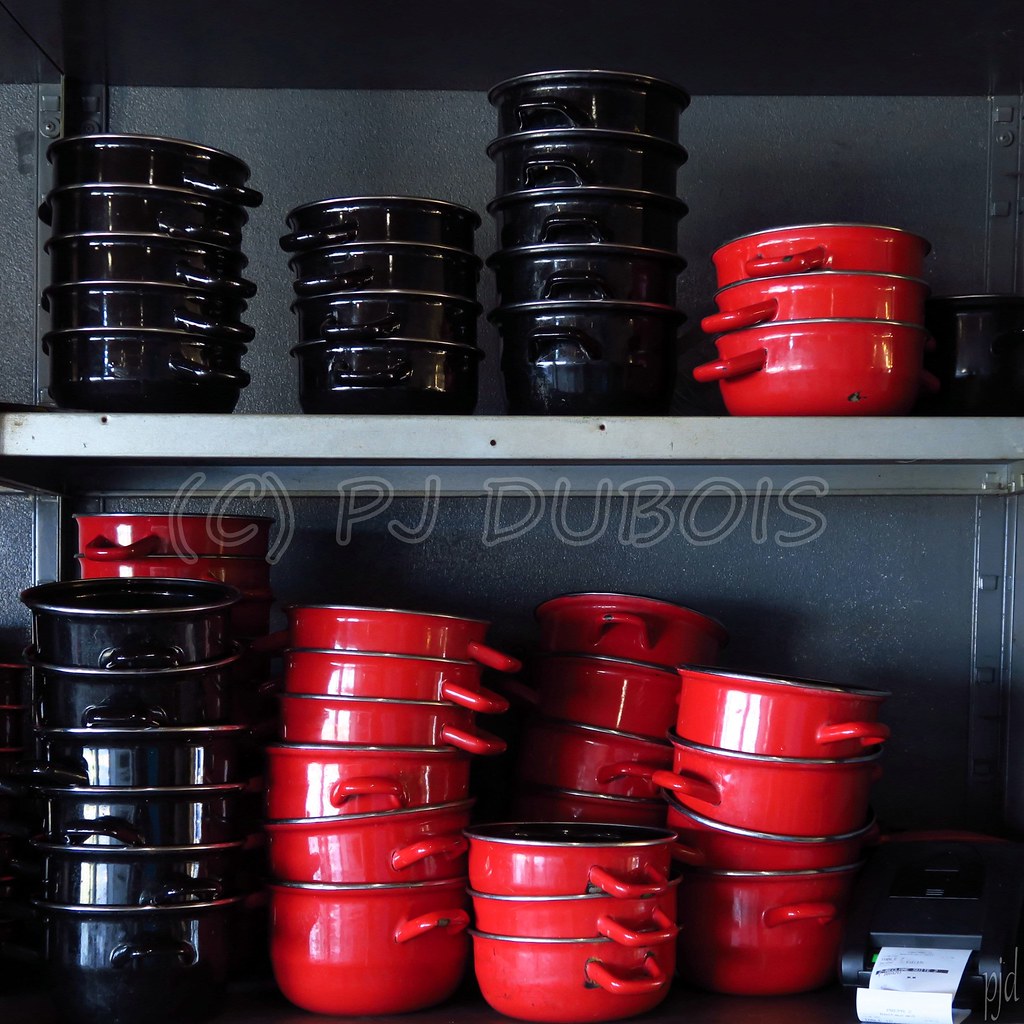This detailed image depicts a neatly organized display of pots and pans, presumably for sale in a store. The shelves are housed within a gray cabinet and each pot is meticulously color-coded and stacked. The top shelf features four neat columns: three consisting of black pots and one of red pots. The black pots are stacked with varying heights, containing five, four, and five pots respectively, each having handles on both sides and a stainless steel interior. The red pots on the top shelf form a slightly wider column with a stack of three.

On the bottom shelf, the color pattern continues with more black and red pots. The left side has a towering stack of six black pots, behind which two red pots are visible. Next, there are six red pots stacked in a single column. Further along to the right, another column of red pots is stacked with three in the foreground and an additional set of three partially visible behind them. The final column on this shelf has four pots. An object resembling a printer or receipt printer is situated in the corner, adding a mundane retail touch to the setting. The entire setup is neatly organized, underscoring a sense of order and symmetry within the cabinet. A watermark on the image indicates © PJ Dubois, signifying the photographer's copyright.